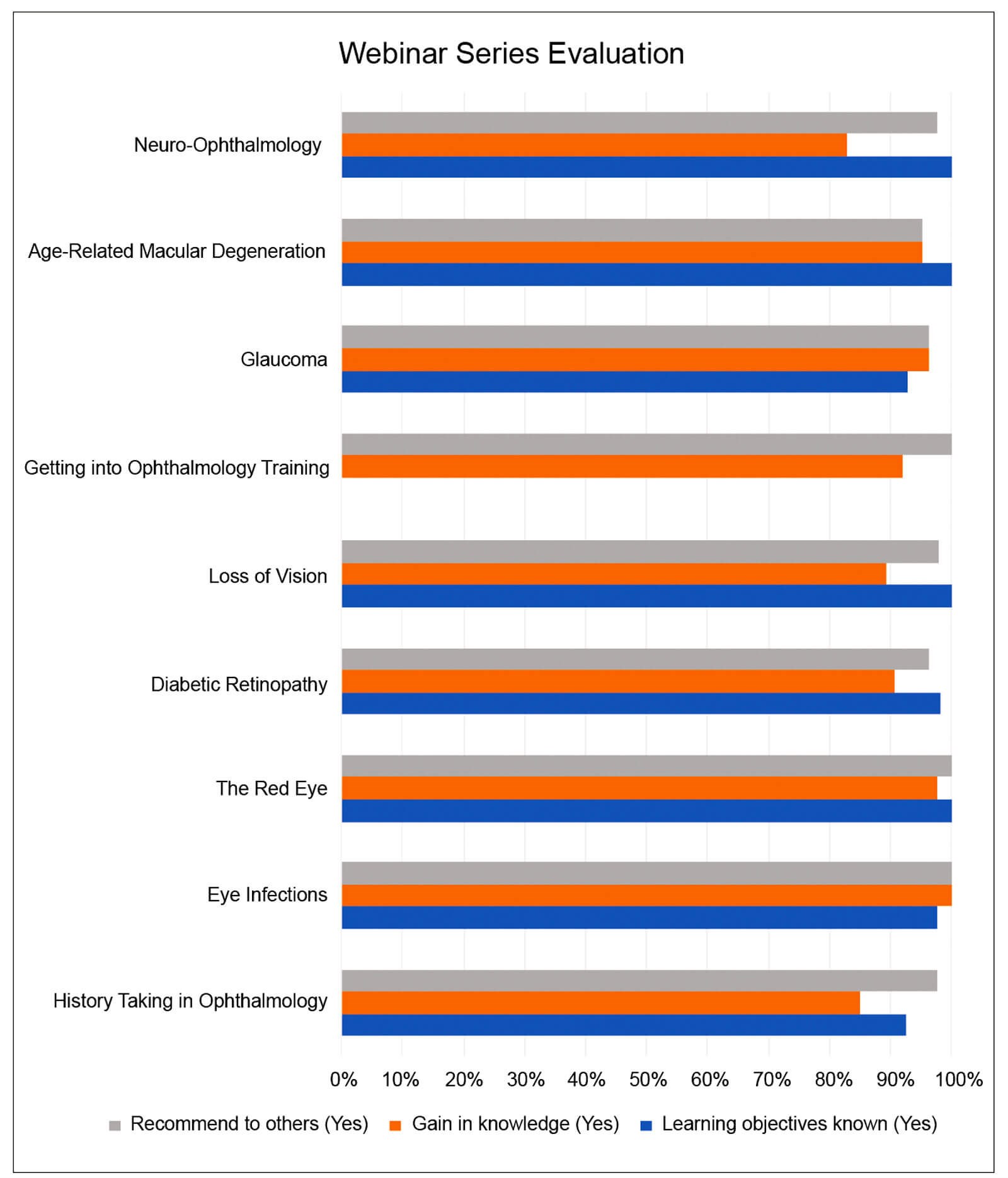This image is a graphic representation of a webinar series evaluation, depicted as a bar graph with values scaled from 0 to 100. The categories evaluated include various medical subjects: age-related macular degeneration, glaucoma, loss of vision, the red eye, eye infections, history taking in ophthalmology, getting into ophthalmology training, neuro-ophthalmology, and diabetic retinopathy. The bars are color-coded to denote distinct evaluation criteria: gray for "recommended to others," orange for "gain in knowledge," and blue for "learning objectives known." The text "Webinar Series Evaluation" is prominently displayed at the top in black. The categories are listed vertically on the left, while the corresponding bars extend horizontally across the graph, illustrating the percentage responses for each criterion.